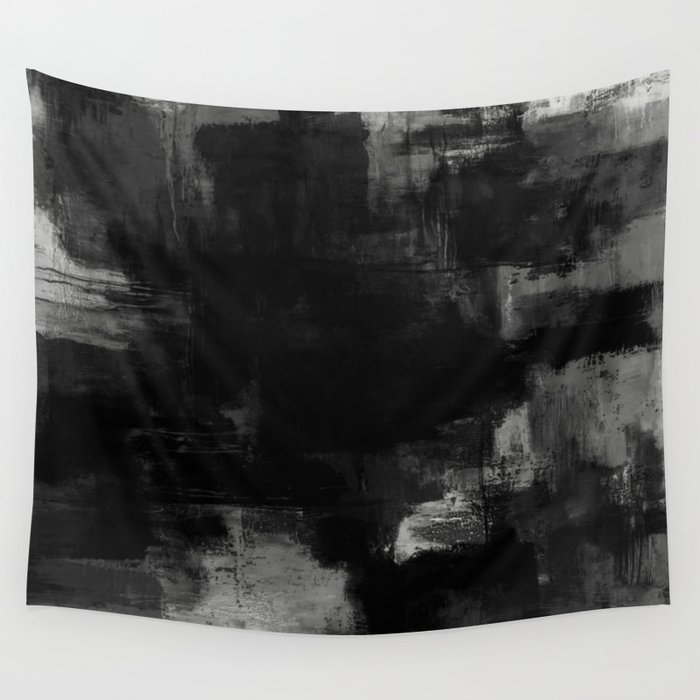In the image, a piece of grayscale artwork is hung against a very light gray background, possibly resembling a bed sheet or piece of canvas. The fabric, slouching slightly in the middle due to the way it's hung, features an array of horizontal strokes and smudges in blacks, whites, and varying shades of gray, creating an abstract, blotchy appearance without a discernible design. The overall aesthetic, perhaps achieved using charcoal or watercolor rubs, conveys a minimalist style. The piece lacks any specific identifiable forms but evokes the texture and feel of an old rusted building. Some lighting from the upper left corner highlights and shadows parts of the fabric, enhancing the depth and texture of the artwork. The background suggests an art gallery setting with a simple white wall, focusing attention entirely on the hanging piece.